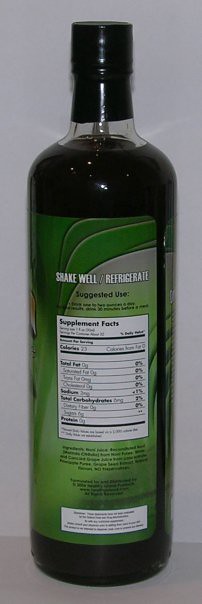This photo features a tall glass bottle with a slender neck, sealed by a black-taped lid. The bottle's label is predominantly green and includes several sections of information. At the top, it advises to "shake well" and "refrigerate," followed by a section on suggested uses, although the specific instructions are too small to be legible. Below that, a white triangle houses the supplement facts, with black text detailing various nutritional information. At the bottom of the label, there's a small rectangle containing additional text, but the details are not clear in the image.